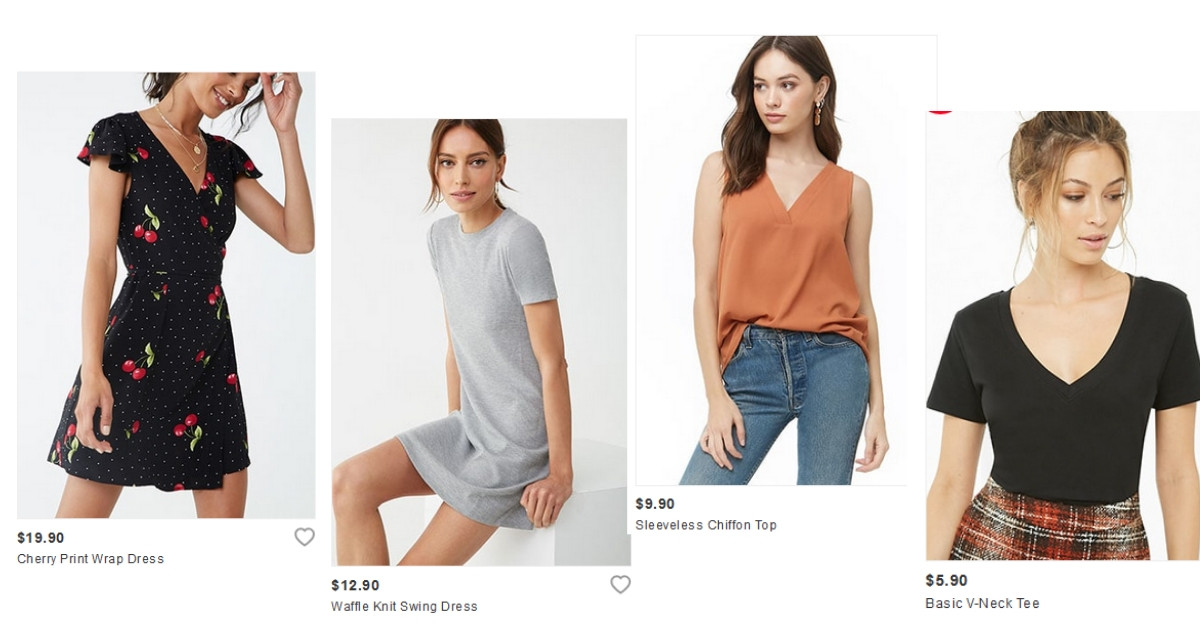The image depicts a webpage of an online retail store, likely akin to H&M or Old Navy, featuring women's clothing against a completely white background. The layout showcases four distinctive clothing items, each within their respective boxes, accompanied by images of women modeling them and product details.

To the left, we see a woman modeling a Cherry Print Wrap Dress adorned with cherry symbols. This dress is priced at $19.90. A heart symbol is present at the bottom right corner of the box, indicating that users can "like" this item.

Next, a Waffle Knit Swing Dress is displayed, featuring a grey color. The model is seated on a white block, showcasing the dress priced at $12.90.

Moving to the right, the third item is a Sleeveless Chiffon Top in orange, paired with blue jeans worn by the model. This top is available for $9.90.

Lastly, a Basic V-Neck T-Shirt, black in color, is shown paired with a red, white, and black plaid skirt. This t-shirt is priced at $5.90.